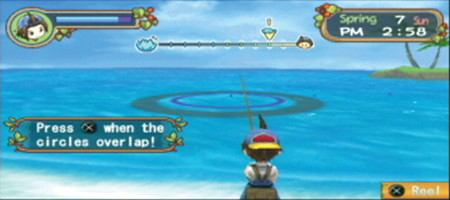In this mobile video game scene, a young boy is seen from behind, leisurely fishing in the middle of the ocean. The setting is picturesque, featuring a tranquil expanse of water under a clear blue sky, with a distant island adding depth to the backdrop. A gameplay instruction hovers on the screen, prompting the player to "Press X when the circles overlap." At the top of the screen, a scrolling bar displays an animated figure of a girl with a pageboy haircut. Additionally, a slider indicates the player's current progress towards capturing an item represented by an acorn. The upper part of the screen contains vital information, including "Spring Sunday 7 PM", with the actual game time displayed as 2:58, suggesting a semblance of real-time progression.